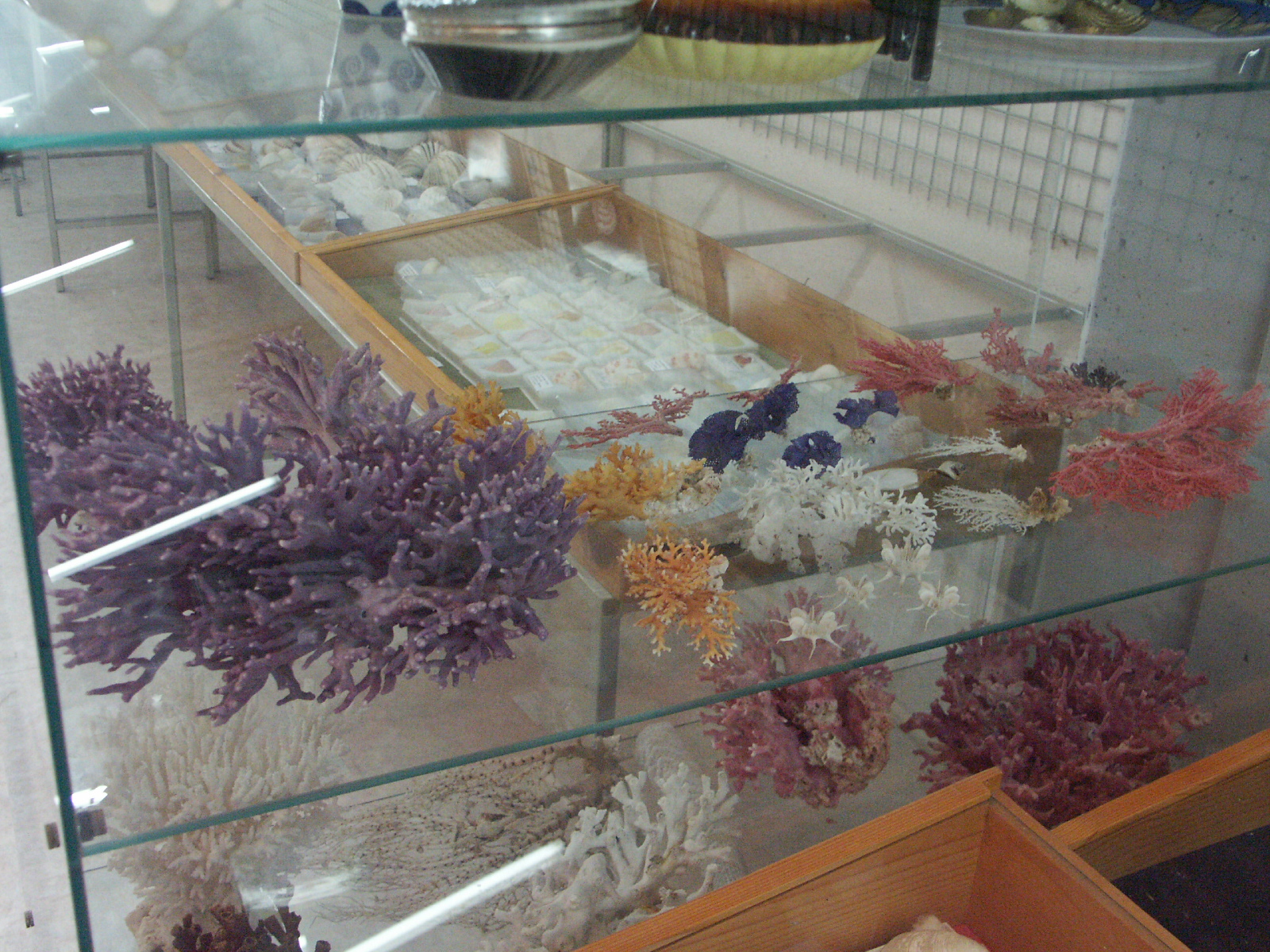The image features a glass display case with three shelves showcasing an array of decorative coral pieces. The top shelf primarily holds various dishware, while the second shelf displays a striking collection of coral, including a large piece of purple coral prominently standing out. Adjacent to it on the left are some orange corals, gradually transitioning to smaller white pieces towards the right, intermixed with occasional red and blue corals. On the bottom shelf, more coral is exhibited: a burgundy-red coral to the right and white and tan corals to the left. In the backdrop, a wooden display case is partially visible, though its contents remain indistinguishable. A metal fixture on the wall, possibly for hanging items, and the corner of a wooden drawer protruding into the foreground suggests the setting is likely a gift shop. The overall color palette of the image includes shades of white, brown, maroon, purple, pink, orange, and occasional touches of gray and yellow, creating a rich, colorful display.